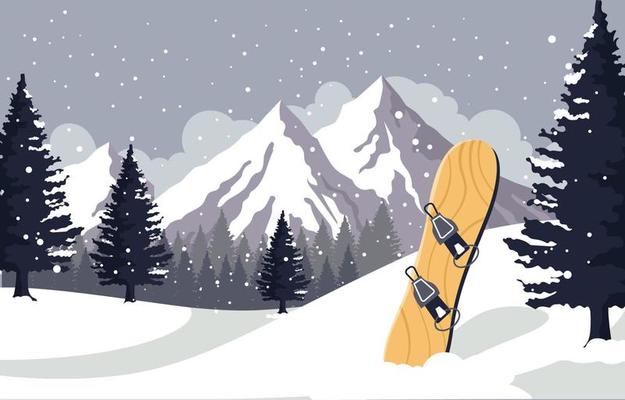This artwork, with a cartoonish style, vividly portrays an outdoor snowy mountain landscape. The ground is covered in white and grey snow, featuring a prominent snowboard standing vertically on the right side, suggesting a potential crash scenario. The snowboard, appearing brown with a wooden grain texture, is equipped with black foot straps. Scattered around the foreground are several pine trees; on the right, a large black tree stands prominent, while other black trees are placed towards the middle and left side of the image. In the background, lighter black and green trees extend towards three snow-capped mountain peaks. The sky is dotted with falling snowflakes, emphasizing the active snowfall in this serene winter scene.